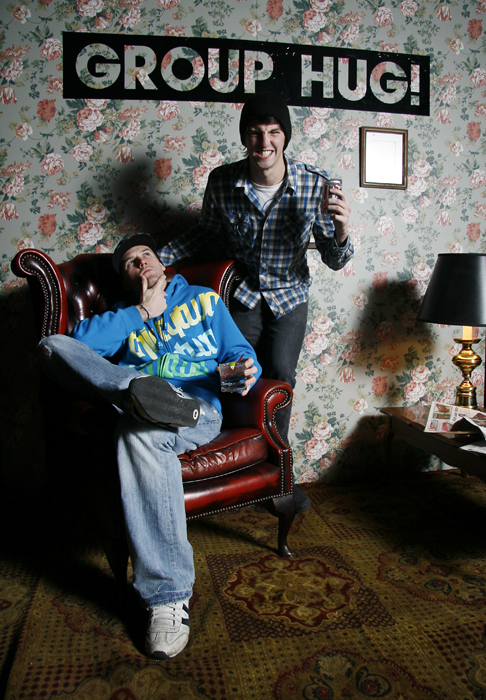In this cozy living room scene, the focal point is a prominent wall sign proclaiming "Group Hug" in a decorative font, encased in a black frame. The backdrop features a sophisticated flower-patterned wallpaper with shades of gray, purple, pink, white, and green leaves interspersed between the letters. Beneath the sign, a picture rests in a brown frame. 

Two individuals appear in the image: one sits comfortably in a red chair with black legs, dressed in a blue hoodie accented with yellow and green, paired with light blue jeans, black and white sneakers, and a black hat while holding a drink. The other man stands nearby, slightly crouched, wearing dark jeans, a white undershirt, and a checkered blue, white, and brown shirt, completed with a black beanie.

To the right, a stylish lamp with a gray top and a golden base casts a shadow against the wall, situated on a brown table. The floor features a green rug adorned with a floral design, harmonizing with the room's decor.